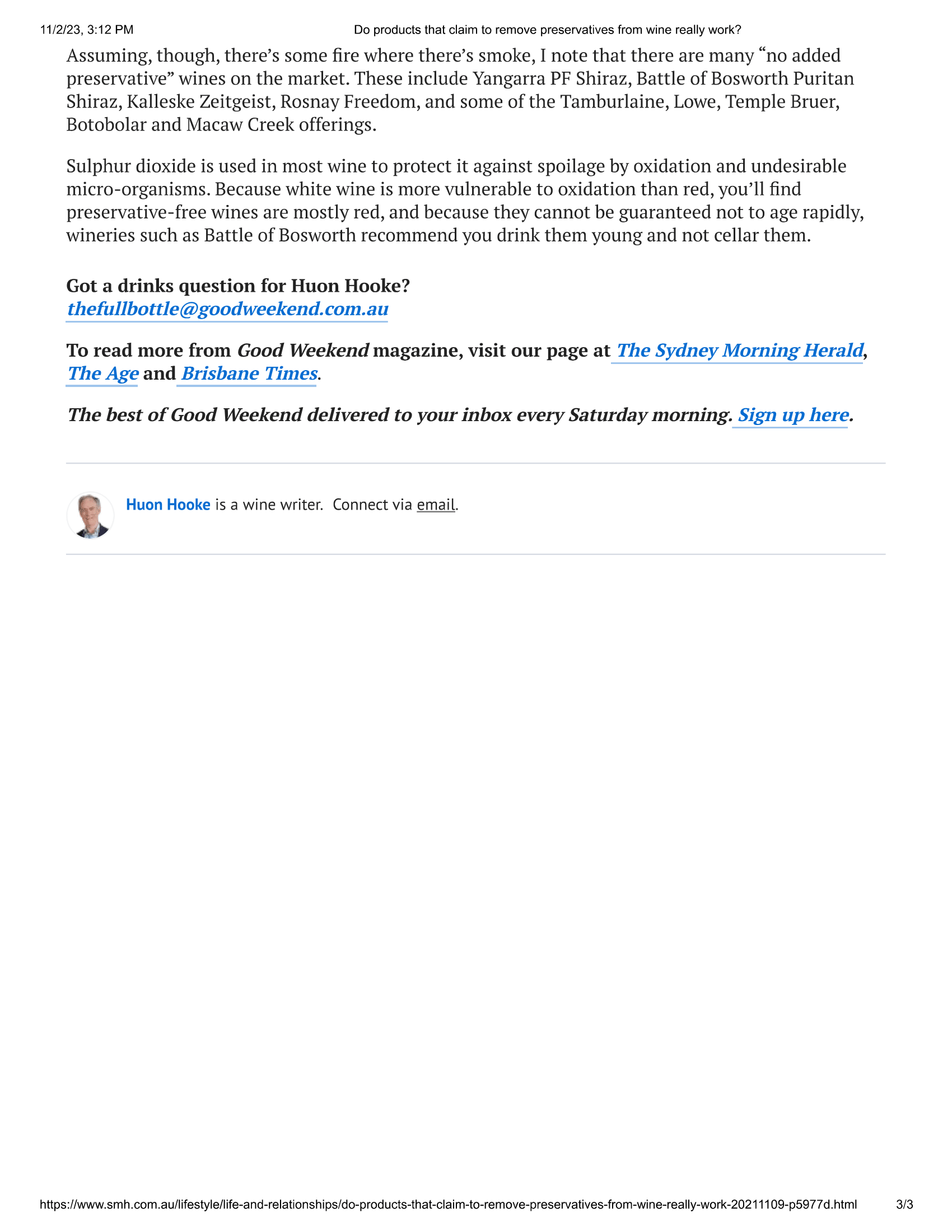The image displays a white background with small black text that is difficult to read, even when zoomed in. The partially legible text underneath the initial sentence seems to discuss the presence of smoke indicating fire. It goes on to list various preservative-free wines available in the market, such as Yungar PF Shiraz, Battle of Bosworth Puritan Shiraz, Kieliski Zilkgeese, Rosne Freedom, Timberlane, Lowe, Temple Brewer, Bata Bolor, and McCall Creek Auburn. The text explains that sulfur dioxide is commonly used in most wines to protect against oxidation and undesirable microorganisms, emphasizing that white wine is more prone to oxidation than red wine. Therefore, preservative-free wines are often predominantly red. It also mentions that because these wines cannot be guaranteed to age well, wineries like Battle of Bosworth recommend consuming them while they are still young rather than cellaring them.